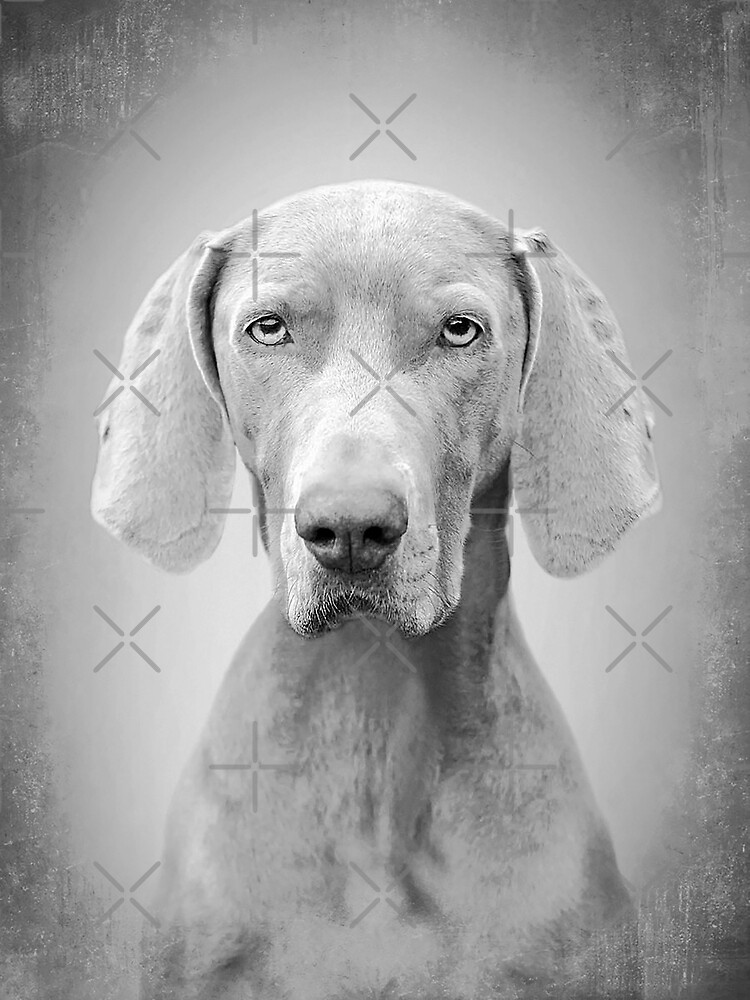This detailed, black and white headshot of a dog captures the essence of a professionally taken photograph. The dog, with a serious and forward-focused gaze, boasts floppy brown ears and a distinct black nose set upon a long snout. The detailed grayscale image highlights the dog's high-definition features, including the individual whiskers on its snout. The composition centers on the dog's face and upper chest, while the background employs a professional blur with a textured border that resembles a grainy stone effect. Adding to the intrigue are light gray watermarks in the shape of X's scattered across the photo. An ethereal circular glow enhances the subject, further amplifying the professional quality of the shot.